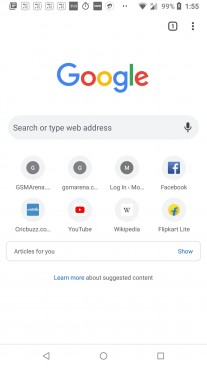The image depicts a smartphone screen with various interface elements. At the very top, there is a status bar displaying multiple icons, including indicators for cellular service, Wi-Fi, a 99% battery charge, and the time, which reads 1:55. Below the status bar, “Google” is prominently displayed in its distinctive multicolored logo: a blue 'G', red 'O', yellow 'O', blue 'G', green 'L', and red 'E'. Directly below the logo is a search bar with a prompt that reads "Search or type your address" and a microphone icon on the right side for voice input.

Beneath the search bar, there is a section featuring various icon clusters and text. The text "G S M A R E N S I" is partially visible, followed by ellipses, suggesting truncated content, then "G M Y E R O", and a "log in" prompt. Next, there is a Facebook icon.

Further down, there are two rows of four app icons each. The first row includes Crickbuzz, YouTube, Wikipedia, and an app labeled Flipart Lite. Below this, a section titled "Articles for you" invites the user to “show” more content, with an option to "learn more about suggested content."

At the bottom of the screen, there is a navigation bar featuring a backward arrow, a circle, and a square. The image quality is poor, making some elements difficult to read clearly.